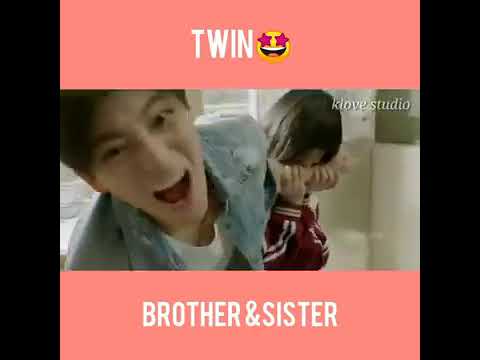The image is a graphic depicting two young men of Asian descent, seemingly captured in a low-quality screenshot that resembles a video frame. The man in the foreground is wearing a blue denim jacket over a white t-shirt, and appears to be yelling or speaking loudly towards the camera. Behind him, slightly to the left, is another man with brown hair styled in a red and white jacket, who seems to be playfully biting the first man's arm. Both men are positioned in the center of the image.

The top of the graphic features a salmon-colored banner with the word "TWIN" in white capitalized letters alongside a yellow smiley face emoji with magenta stars for eyes. Identical emojis with stars for eyes are positioned in both the top and bottom banners. Below the image, a similar salmon-colored banner displays the words "BROTHER AND SISTER" in white text. The name "Clove Studio" is noted in the top right corner of the image, indicating the likely source. The background of the image is slightly blurred, showing a room with white walls and windows with blinds through which light is streaming in. There are also small vertical black banners on the left and right edges of the image.